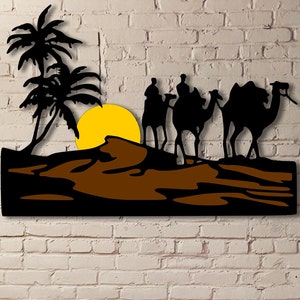The image features a decorative art piece mounted on a creamy white painted brick wall. This artwork is crafted in a stenciling or cut-out style using an unidentifiable material. It depicts a desert scene with a dark brown sandy hill featuring black shadow outlines that form peaks and valleys. In the upper left corner of the piece, two black silhouette palm trees are situated: one mostly upright and the other angled slightly to the side. Just above the sand, to the left of center, a bright yellow sun is partially visible. Situated to the right of the sun, three camels are depicted in silhouette, traversing the sandy terrain. Two camels, closer to the sun, have indistinct figures riding them, while the largest camel, located further to the right, carries a large pack on its back but has no rider. The entire scene is rendered in stark silhouettes, giving it a striking visual contrast against the white brick background.